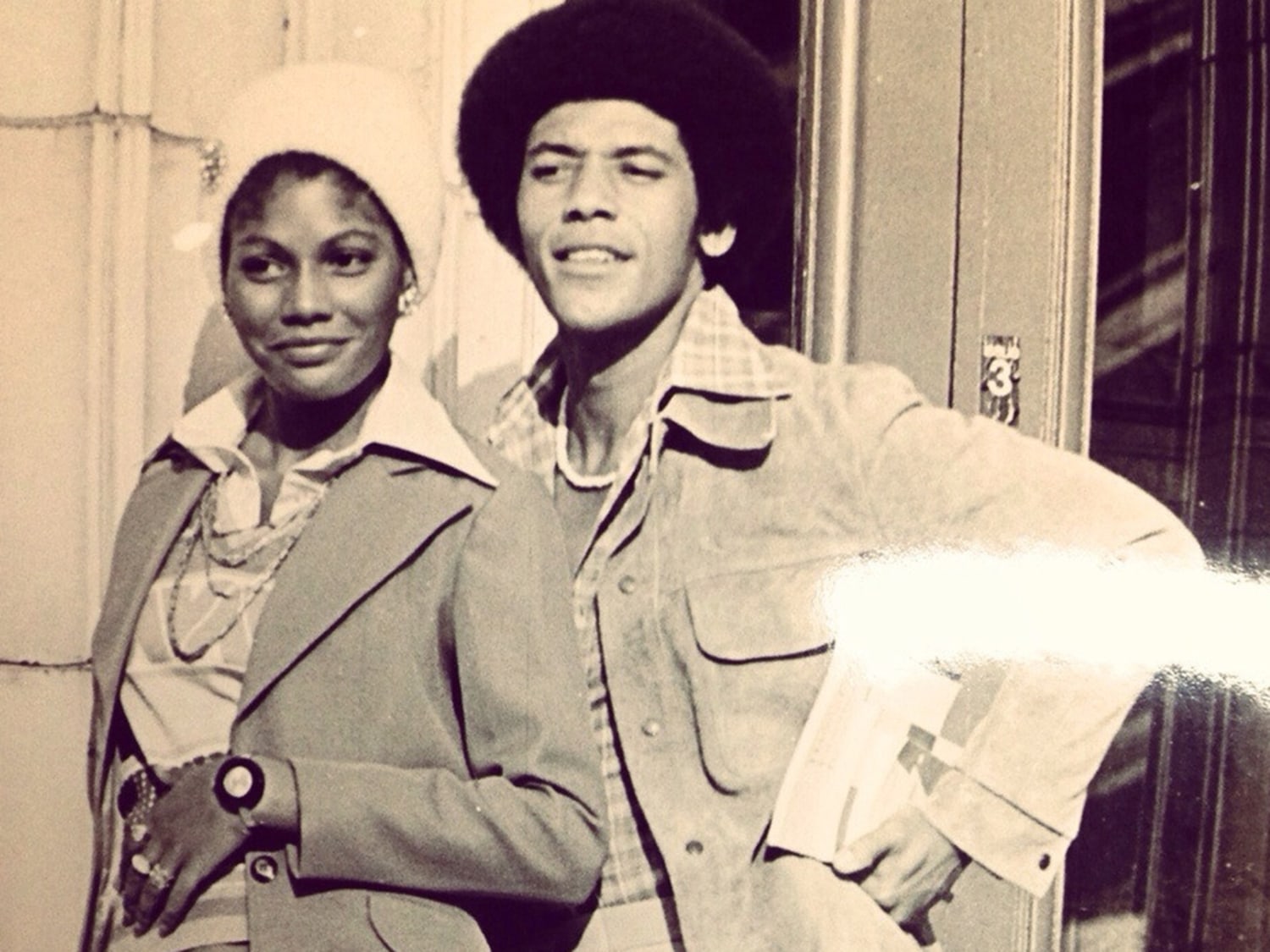This is a vintage black-and-white photograph, likely from the 60s or 70s, with a slight sepia tinge due to age. The image is rectangular and longer horizontally than vertically, capturing an African American couple standing in front of a door marked with the number three. On the left side of the photograph is the woman, who is smiling and wears a white hat with a pin, earrings, a gray jacket, and a blouse with an upturned collar over the jacket. She has three necklace chains and jewelry on her wrist and hand, with her left hand resting on her stomach. Her hair is either short or tucked under the hat. To her right stands the man, slightly behind her, also smiling. He wears a plaid shirt with a large pocket and flap, a jacket similar to the woman's, a white necklace possibly made of seashells, and has an afro. Tucked under his left arm, he holds an indistinguishable object, possibly a magazine. The right side of the photograph has a darker black area with some glare approximately two-thirds of the way down. Both individuals are looking slightly toward the left, and their clothing styles reflect the vintage era of the 70s.